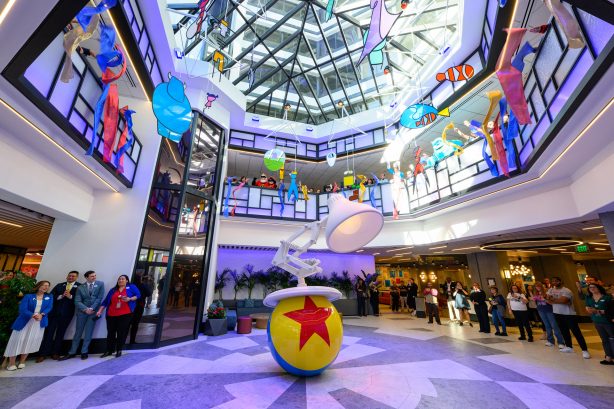The image captures the interior of a large, multi-story mall, distinguished by a striking glass roof that illuminates the space. Central to the scene is a grand sculpture featuring a substantial, yellow and blue ball adorned with a prominent red star. Perched atop this ball is an oversized white lamp, reminiscent of a reading lamp, which arcs gracefully and seems proportionally as large as the ball itself. Surrounding this intriguing centerpiece, numerous people can be seen, some dressed in suits with lapel ID badges, suggesting a professional gathering or special event. Many individuals are actively taking pictures, hinting at the sculpture's popularity or significance. 

The mall's second floor, bordered by a glass railing, showcases vibrant decorations, including banners, pennants, and a whimsical mobile suspended from the ceiling. The mobile features colorful orange and blue fish along with other playful, toy-like creatures that add an element of whimsy to the setting. The floor beneath is a pattern of purple and white marble, enhancing the elegance of the space. Additionally, small shrubs appear in the background, adding to the decorative ambience. The overall scene suggests a lively and engaging environment, potentially the site of a special event or art installation.